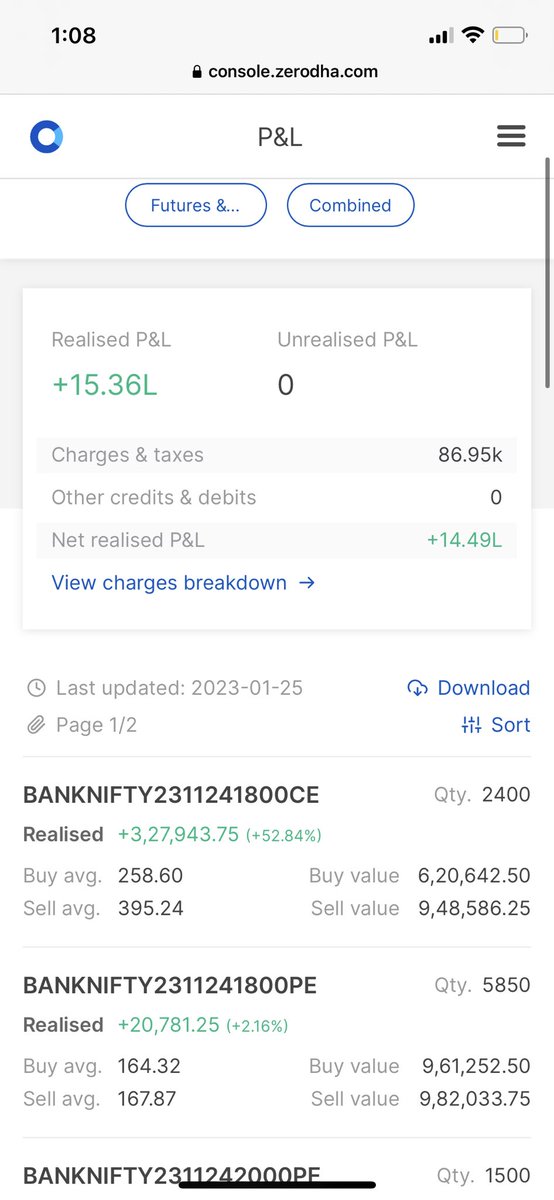**Detailed Caption:**

The image is a screenshot of a smartphone displaying an app. The status bar at the top of the phone screen indicates the time as 1:08, along with icons for cellular signal strength, Wi-Fi, and battery status; the battery is low and shown in yellow. The website currently open in the app is "console.0dha.com."

In the top left corner of the website, there is a blue circular logo with "P&L" in the center. To the right of the logo, there are three horizontal lines indicating a menu option. Beneath these elements, the website displays a blue tab with rounded edges labeled "Futures" and an ellipsis ("...").

Further down, there are detailed financial statistics:
- **Realized P&L:** +15.36L
- **Unrealized P&L:** 0
- **Charges and Taxes:** 86.95K
- **Other Credits and Debits:** 0
- **Net Realized P&L:** 14.49L

A blue font link, "View charges and breakdown," accompanied by an arrow, is shown beneath these statistics. It also states, "Last updated 2023-01-25," "Page 1-2," and includes options to "Download" and "Sort," which are colored in blue, while all other fonts are gray.

Further down, the image lists financial details for "Bank Nifty 2311241800CE" and directly below it "PE," each accompanied by information about quantity, buy average, sell average, buy value, and sell value.